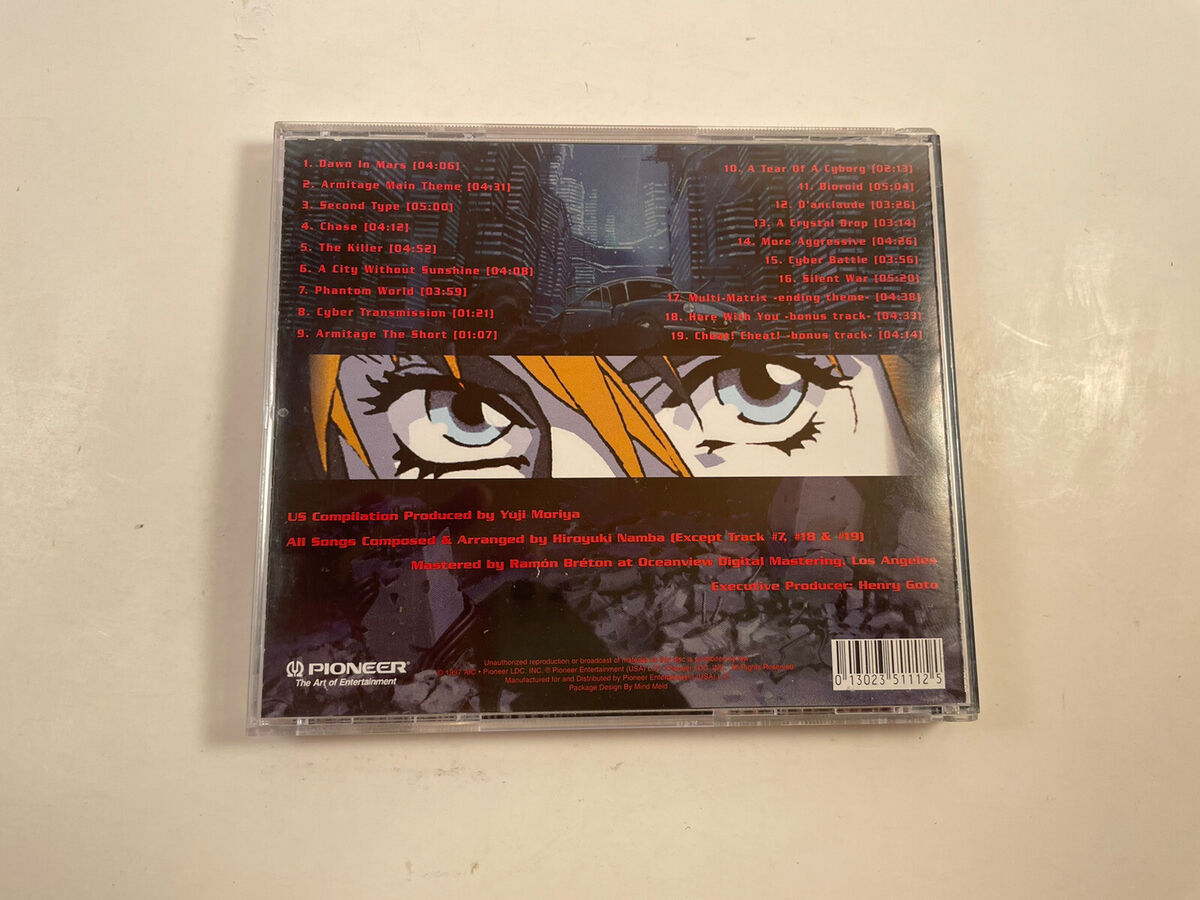This detailed image captures the back cover of a CD jewel case. The cover features a striking blend of imagery and information. Dominating the design is a vividly animated graphic, characteristic of Japanese anime, showcasing a section of a woman's face with large, blue, expressive eyes framed by blonde hair. Her facial features are set against a backdrop that depicts a dark, underexposed futuristic cityscape with towering buildings, and scattered concrete debris or trash at the lower third of the image. 

This animated face is divided by a horizontal banner running through the middle of the background. The image is further enriched by a small car cruising along the futuristic cityscape, adding to the dynamic visual storytelling.

The listing prominently displays 19 song tracks numbered in red text. While the exact titles of most tracks are not clearly legible, mentioned songs include "Down to Mars," "Second Type," "Chase," and "The Killer." Each song's length ranges from one to five minutes. The tracks are noted to be mostly composed and arranged by Hiroyuki Namba, with exceptions for track numbers 7, 18, and 19, which are produced by Yuji Moriya.

Additional details include a Pioneer logo positioned on the left with the phrase "the art of entertainment" beneath it and an ISBN number located at the bottom right corner. This well-composed image not only provides a comprehensive listing of the CD content but also captures the thematic essence of the animations and cityscape.